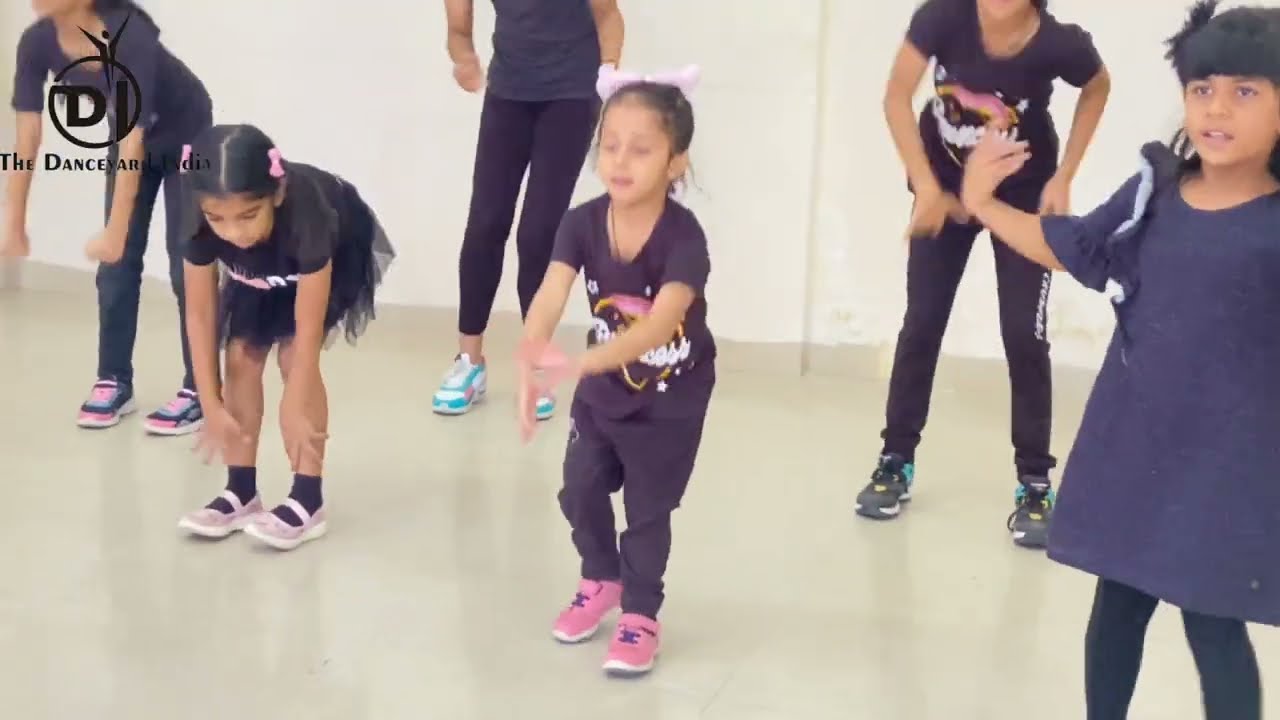The image captures a dynamic moment in a dance class featuring six girls of varying ages, all engaged in different dance movements. Toward the front are three young girls, each distinct yet uniformly dressed in black attire with consistent details like bows and printed graphics. The girl on the far left is leaning over with her arms extended downward, sporting black and pink shoes. To her right, a smaller girl reaches toward her toes, wearing a black dress and pink shoes. The third girl, taller and positioned at an angle, wears blue and white shoes.

Behind them stand three older girls, possibly teenagers or adults, also mid-movement, suggesting a choreographed performance. One of them is wearing a T-shirt with the word "Princess" printed on it and sports a bow in her hair and pink shoes. The next girl, leaning forward with her arms extended, echoes this with a similar "Princess" T-shirt and black and blue shoes. Finally, the girl on the far right is adorned in a dark blue dress with frills on the shoulders, her hand outstretched and eyes focused to the left.

The scene is set in a dance studio with a shiny, light brown floor and a cream-colored wall. At the top left corner of the image appears a logo featuring a black circle with a 'D' and an 'I', accompanied by a small, triangle-shaped figure with raised arms, and the text "Dance Yard India" below it. The cohesive attire, shared dance movements, and studio setting convey a focused but lively atmosphere.